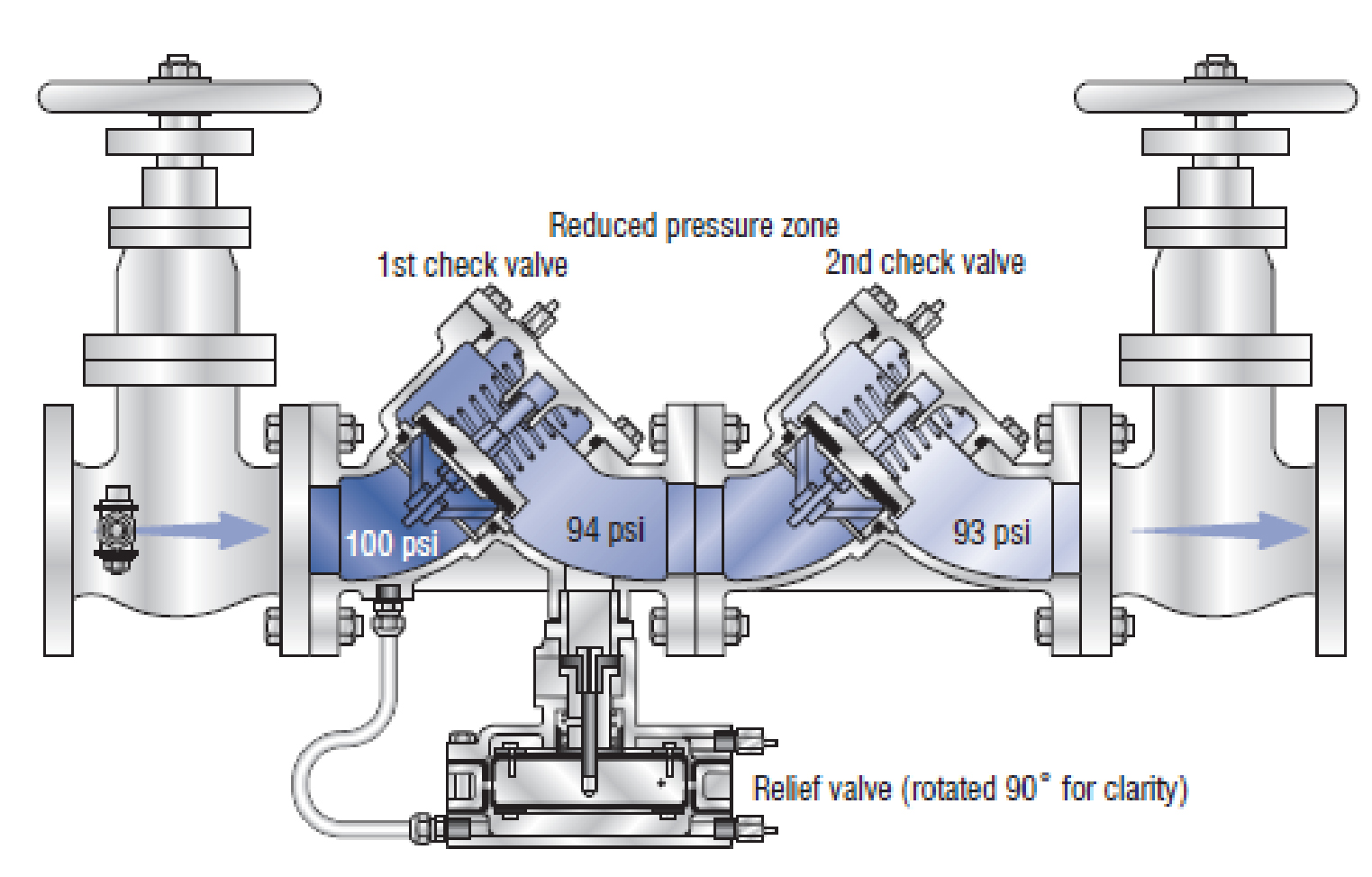The image displays a detailed diagram of a mechanical structure, likely a valve or pressure pipe system. The entire structure appears to be primarily silver-colored with some gray and white accents, set against a white background. The diagram highlights important components and areas using labels. At the top, there are two circular knobs or wheels on the left and right sides. Labels at the top read "First Check Valve" on the left and "Second Check Valve" on the right, both in blue text. The central section features a "Reduced Pressure Zone" label, signifying a specific area within the structure.

Flowing through the tube, blue water can be seen with pressure readings of "100 PSI" on the left side, "94 PSI" in the middle, and "93 PSI" further to the right. Blue arrows indicate the direction of flow towards the right side of the diagram. At the bottom, a component labeled "Relief Valve" is annotated with "(Rotated 90 degrees for clarity)" also in blue text. Beneath the pipe, there's an additional mechanism, which could be a pump, associated with the relief valve. Alongside this, another blue arrow points right. Moreover, notable tools or fasteners such as bolts, nuts, or screws are present, particularly to the left of the pipe. Overall, the image meticulously illustrates the components of a pressurized piping system with clear labels and flow directions.